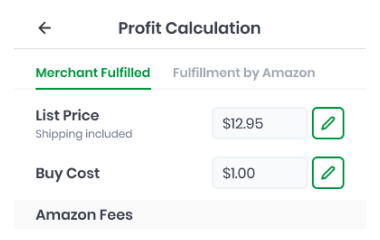The image features a white background with a detailed illustration of a profit calculation process. At the top, an arrow pointing to the left is labeled "Profit Calculation" in blue text. Below the arrow, a thin blue line separates the sections.

"Merchant Fulfilled" is written in green text, underlined for emphasis, while right next to it, "Fulfillment by Amazon" appears in light blue text. These two options are central elements of the illustration.

There is a prominent list price indicated by a blue box containing the value "$12.95," situated next to a small green box with a green pencil icon inside it. Below this, the term "Buy Cost" is displayed, accompanied by a blue box showing the value "$1" and another green box featuring a green pencil icon. Further down, another blue box is labeled "Amazon Fees", although the fees are not explicitly detailed in the image.

This visual representation succinctly outlines the components involved in calculating profit, distinguishing between merchant fulfillment and Amazon's fulfillment options, along with price points for list price, buy cost, and an unspecified section for Amazon fees.